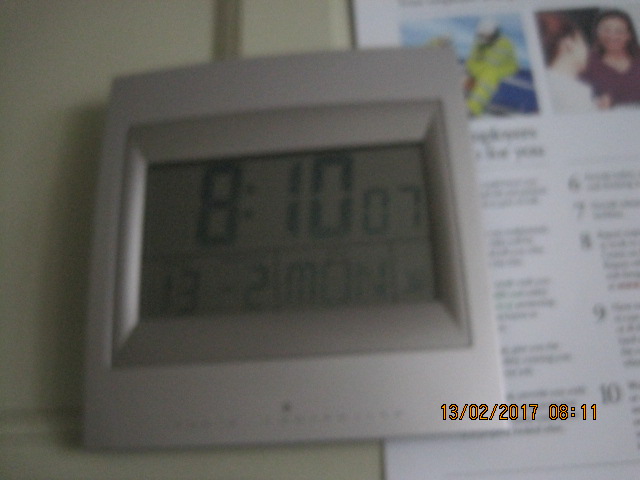The image depicts a digital clock housed in a gray-framed casing, though the entire photograph is notably blurred. The primary display of the clock shows the time as 08:10:07. Below the main time display, there are additional numbers or information, though they are indiscernible due to the blur. The clock rests on a gray-colored surface. Occupying the right side of the image is a white sheet that features a layout of people in small squares at the top, indicative of a video call or conference, followed by rows and columns of text below. In the lower right-hand corner of the photograph, a red time stamp reads "13-02-2017, 08-11."